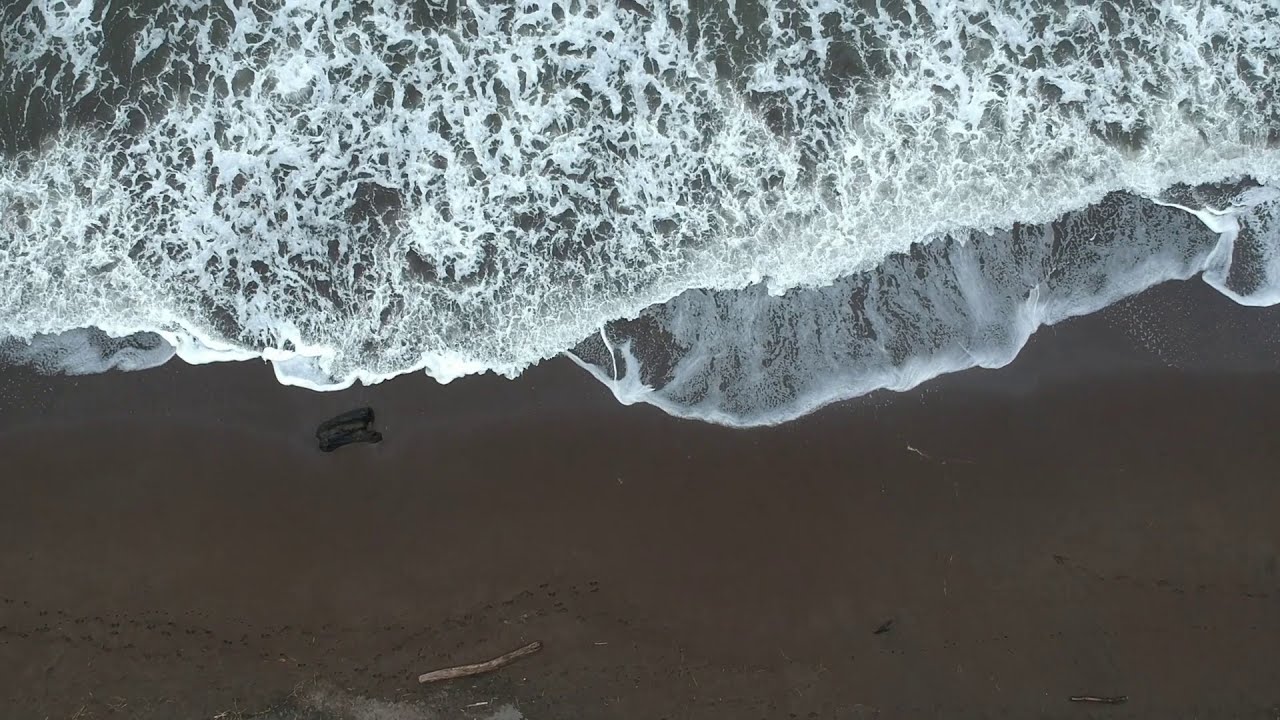This full-color aerial photograph, captured by a drone, offers a bird's eye view of a shoreline during the daytime. The image reveals a dynamic beach scene where the ocean's waves crash onto the shore, creating a striking contrast between the foamy white surf and the aquamarine water. The dark brown, wet sand occupies the bottom half of the photo, decorated with a few footprints and pieces of driftwood. Notably, there's a smaller, darker piece of driftwood closer to where the waves reach, and at the bottom center, a lighter-colored stick stands out. The waves form intriguing patterns, with one section resembling a tongue shape as it extends towards the shore, and swirls are visible on the left side of the photograph.